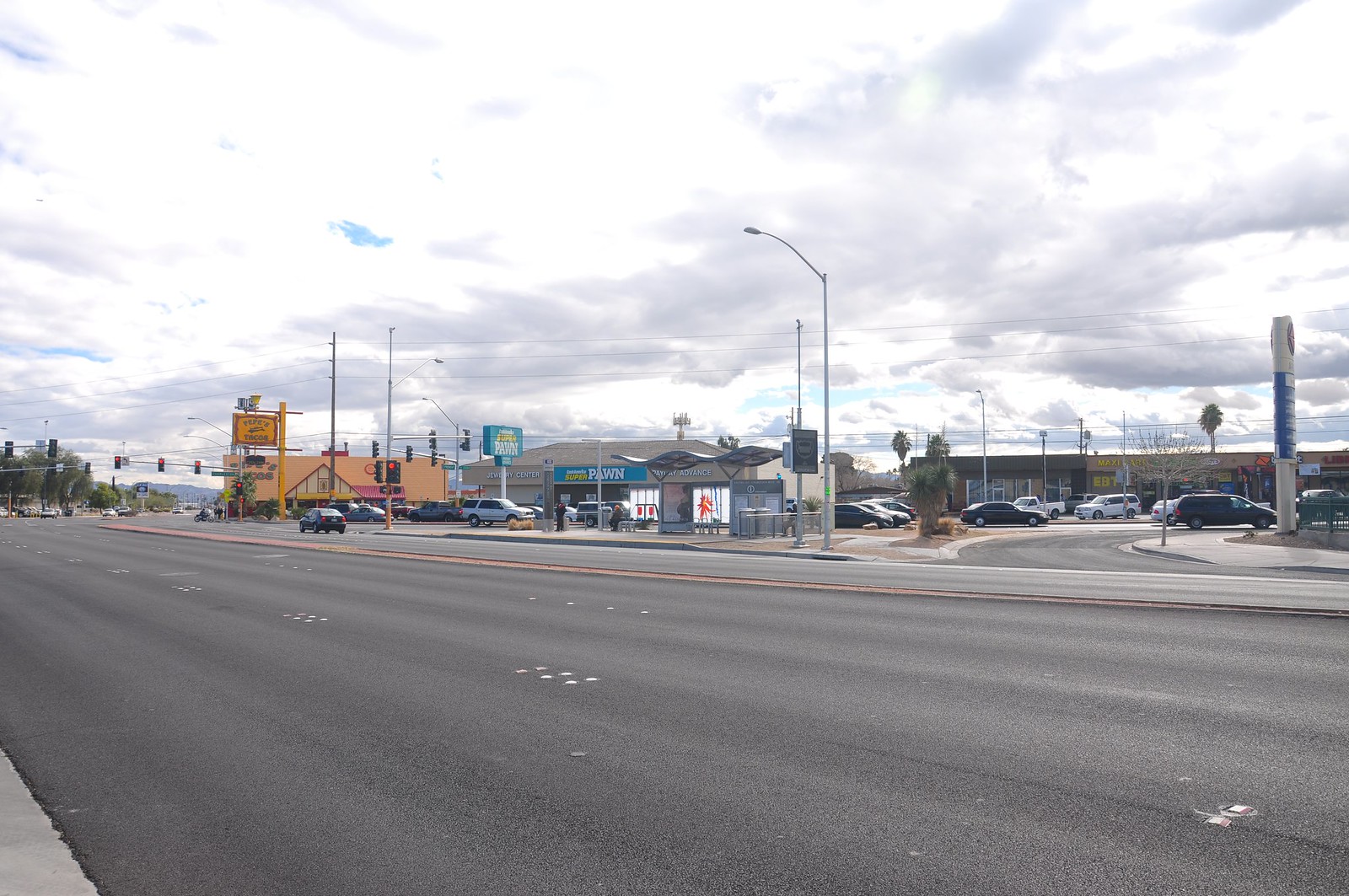The photograph captures a dynamic urban scene with a distinct division between the sky and the earth. The top half of the image showcases a dramatically cloudy sky, filled predominantly with puffy white clouds. Occasionally, patches of vibrant blue sky pierce through, adding a touch of color to the otherwise overcast atmosphere.

In sharp contrast, the bottom half of the image features a bustling road which winds from the bottom right corner of the frame to the middle left area. Alongside, a collection of eclectic buildings and businesses stretches across the horizon. From left to right, the visual journey begins with an orange building bearing a prominent billboard that boldly reads "Pepe's Tacos." Adjacent to it, a tan building comes into view, possibly labeled "Avery Center," followed by a blue sign advertising "Super Pawn," complete with its own billboard. Continuing rightward, the sequence culminates with another building partially hidden by a nearby bus stop, which appears to carry a sign reading "Something Advance."

Further to the right, the scene includes a parking lot, situated behind which lies another strip of small businesses. Though these shops are too distant for their names to be discerned fully, one clearly features an "EBT" sign, while another proudly displays the "Boost Mobile" logo. Notably, standing slightly in front of this array is a gas station price board sign, grounding the busy, layered, and vibrant composition of this urban landscape.